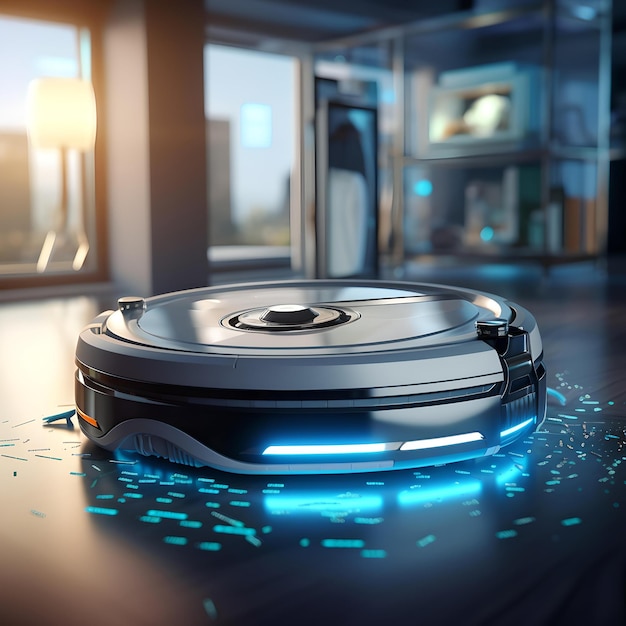This vertical rectangular image captures a close-up view of a robotic vacuum, specifically a Roomba, set against a smooth, hardwood floor strewn with small pieces of paper or confetti. The vacuum is predominantly grey on top with a black bottom edge, and features blue and white lights that highlight the debris on the floor. Central to the design is a circular button on top, flanked by additional buttons on either side. The scene is illuminated by a combination of natural sunlight streaming through floor-to-ceiling windows and artificial light, enhancing the warm tones of the wooden floor. In the blurred background, on the upper left, a brass lamp with a white lampshade can be seen sitting on a windowsill, while the upper right reveals shelves stocked with various products, possibly indicating that this setting could be an art gallery or a retail space. The overall ambiance of the photograph is modern and well-lit, emphasizing the sophisticated design of the vacuum.